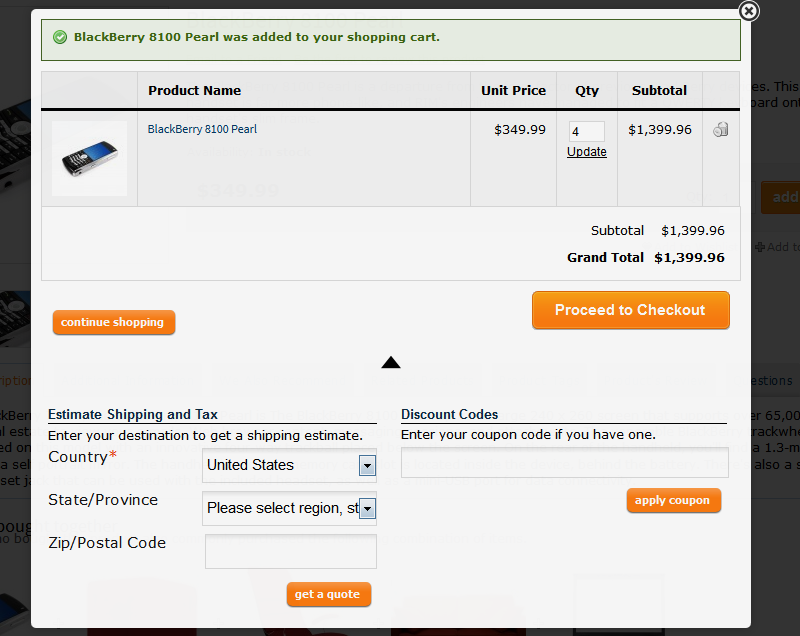The image features a dark black background, primarily overlaid by a large gray pop-up window. At the top of this window, there's a noticeable green rectangle displaying the message: "BlackBerry 8100 Pearl was added to your shopping cart."

Below this message are sections labeled in black text: "Product Name," "Unit Price," "QTY" (Quantity), and "Subtotal." In the subsequent blue text, the item "BlackBerry 8100 Pearl" is listed, followed by detailed pricing information:

- Price per unit: $349.99
- Unit quantity: 4
- Total price: $1,399.96

At the bottom of the itemized section, the text specifies the "Subtotal" as $1,399.96 and the "Grand Total" also as $1,399.96.

Below these details, there's an orange rectangle with white text that reads "Proceed to Checkout." Adjacent and slightly beneath this, another orange rectangle, also with white text, says "Continue Shopping."

Further down, a section titled "Estimate Shipping and Tax" invites users to enter their destination details for shipping estimates. It includes fields labeled:

- "Country" (an entry marked with a red asterisk, indicating "United States" is already selected)
- "State/Province" (displaying "Please select region, ST")
- "ZIP/Postal Code" (currently left empty)

An orange button labeled "Get Quote" is located next to these fields.

At the bottom, there's a section titled "Discount Codes," prompting users to "Enter your coupon code if you have one."